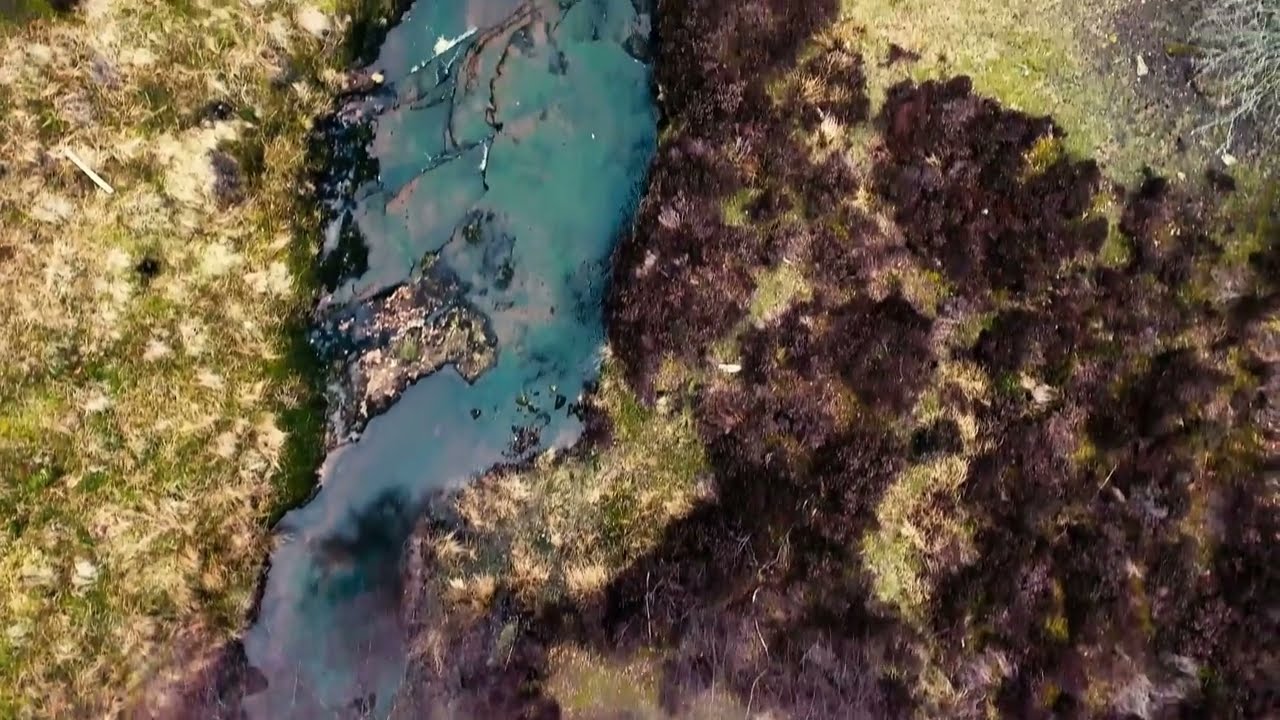This is a high-resolution drone photograph captured from approximately 50 feet above a murky, potentially frozen lake. The top-down view reveals intricate details of the surrounding landscape, painting a somber, almost melancholic scene. The lake itself dominates the center of the image, its water a disturbing mix of green and brown hues, likely contaminated with oil, giving it a greasy, reflective surface that's both blue and blackish in areas.

To the right of the lake, there's a stark contrast of dark brown, dead plants interspersed with patches of yellowish-white dead grass, indicating the withering effects of winter or fall. This section appears particularly barren, with spongy, decayed vegetation suggesting possible oil damage. On the left side, you see a blend of grass and reeds, scattered amidst healthier-looking patches of green. Towards the upper left, the grass appears more vibrant.

Overall, the imagery hints at an environment struggling under the weight of seasonal change and pollution, with the forested right side of the image opposing the more sporadic grassy sections on the left, all unified by the common theme of deterioration and decay.